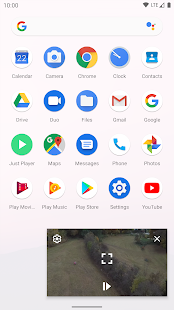The image appears to be a detailed snapshot of someone's mobile phone homepage. At the top left corner, the time is displayed as 10:00. On the top right, there are several status icons: a Wi-Fi symbol, LTE indicator, a partially filled triangle signifying cell signal strength, and a fully darkened battery icon indicating battery life. Below, there's an oval-shaped Google search bar with a 'G' logo.

The main section of the screen showcases a grid of application icons organized alphabetically in four rows and five columns. The icons start from the upper left: "22" labeled as Calendar, followed to the right by icons for Camera, Chrome, Clock, and Contacts. This pattern continues, ending with YouTube at the bottom row's end.

Beneath the application icons, there is a blurry black and white image that seems to depict a video. The image includes a play arrow symbol and an 'X' to close it, suggesting it might be a screenshot of a video rather than an actual embedded video on the screen.